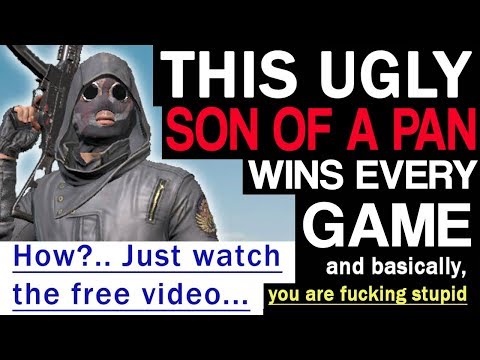This image appears to be a thumbnail for a video or advertisement, possibly designed for a platform like YouTube. The top and bottom of the thumbnail are bordered in black. At the center-left stands a 3D-rendered video game character, visible from the chest up. This character is outfitted in a black leather jacket with a high collar and a hood pulled up over their head. Their face is obscured by a mask featuring black circular lenses and an open mouth, and they wear black fingerless gloves. The character is holding a submachine gun, with the barrel pointed upwards.

The prominent and somewhat provocative text on the right side of the image reads, "This ugly son of a pan wins every game and basically you are fucking stupid." The phrase "son of a pan" is highlighted in red, while "you are fucking stupid" appears in yellow and is underlined. The rest of the text is in white. Below this text, there's an additional line in blue that says, "How? Just watch the free video." 

The overall design suggests an effort to attract viewers through bold, eye-catching colors and controversial language, targeting an audience likely interested in gaming content.